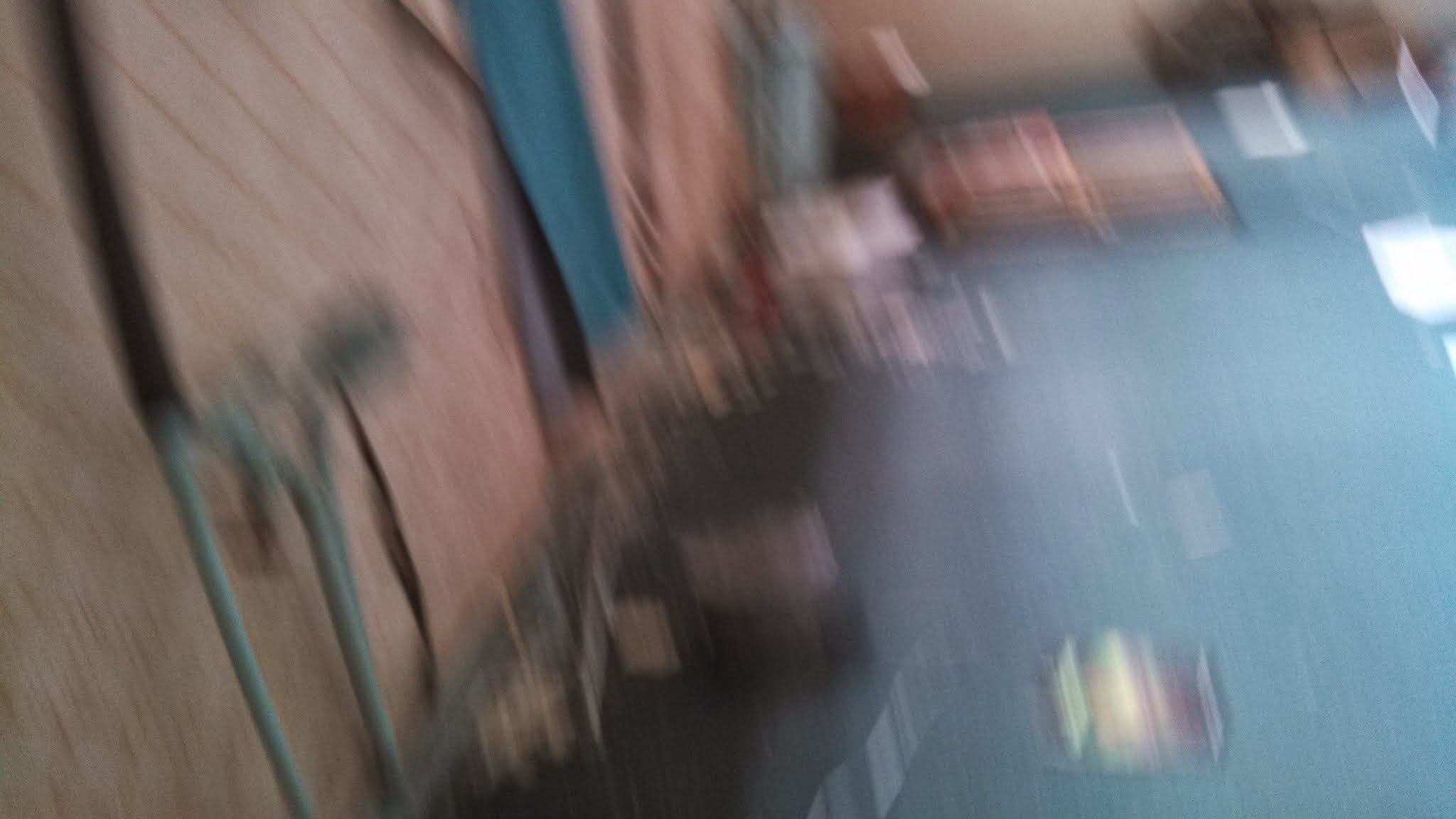This blurry image features a predominantly teal color palette, with various hues ranging from light to dark teal. A piece of cloth in a darker teal shade appears to hang on the wall, contributing to the overall ambiance. The surface, possibly wood, showcases light to medium brown tones with a hint of reddish shade, adding an organic touch to the scene. Metallic elements are discernible in the lower left corner, reflecting light and adding a subtle gray, green, black, and white spectrum to the mix. At the upper right, there are indistinct shapes that could be steps or seating, though the exact nature is obscured by the blur. The floor is a gradient of light to medium teal, aligning at a 45-degree angle from the top left to the bottom right of the image. Reflections from a light source further diffuse across the composition, making it difficult to pinpoint specific details but enhancing the overall ethereal quality.